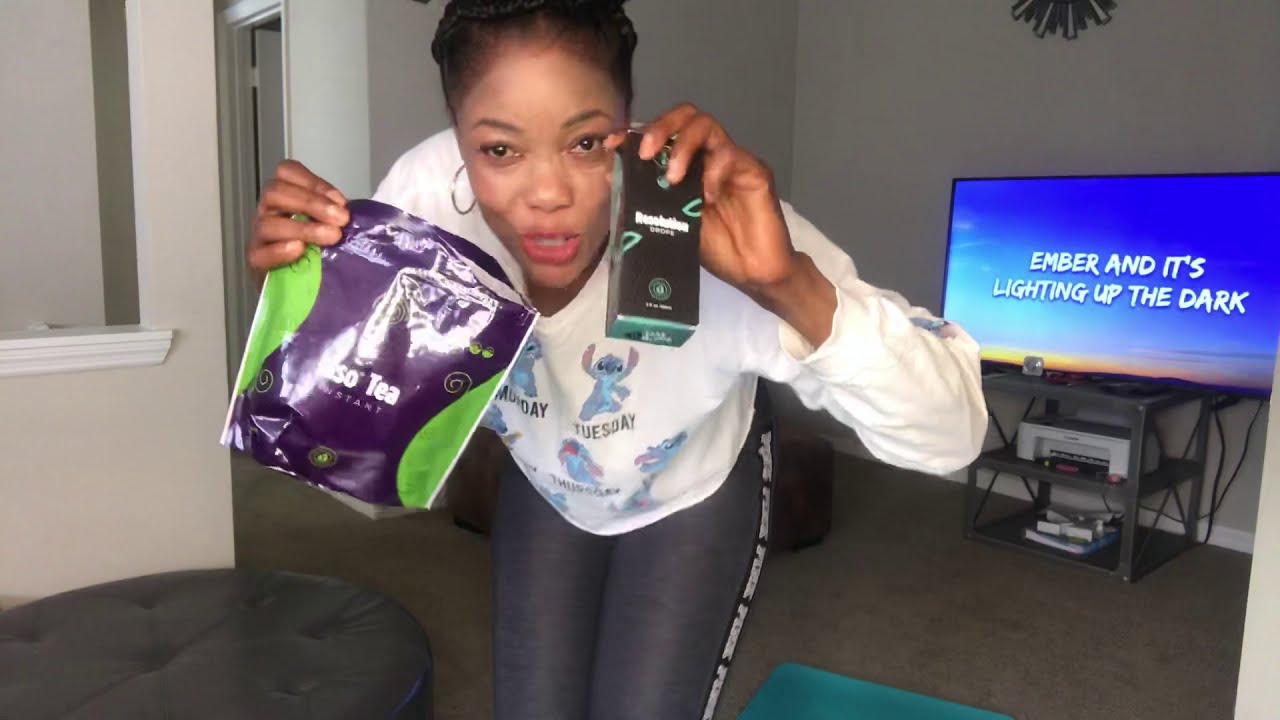This is a horizontal rectangular photograph of an African American woman with black hair, either short or pulled back, bending slightly while holding two items. In her right hand, she holds a purple and green bag of tea, partially obscured by a reflection but clearly displaying the word "tea." In her left hand, she holds a small black and green rectangular box, possibly a product with the word "drops" on it, though the details are hard to discern. She is speaking to the camera, mouth open slightly, and is adorned with silver hoop earrings. Her attire includes a long-sleeved white shirt featuring a cartoon character and the days of the week, paired with gray leggings. The setting appears to be a living room, identifiable by the white or gray walls with white baseboards, and brown carpet. In the background to her right is a TV stand with a TV screen displaying the words "Ember," and "it's lighting up the dark." Additional furnishings include a footstool in the lower left-hand corner and possibly a workout mat nearby.